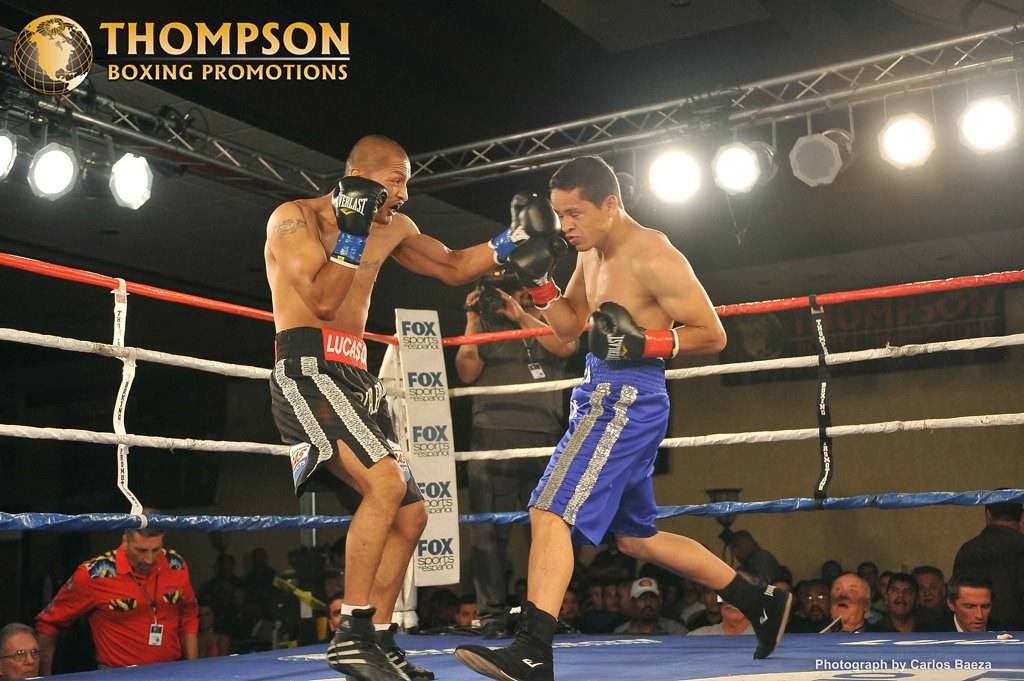In an indoor, color photograph capturing a lively boxing match, two men are locked in combat within a well-lit ring. On the left, a boxer with brown skin and a shaved head, clad in black and white trunks with "Lucas" inscribed on his waist belt, delivers a punch with his left arm. He is also equipped with black boxing gloves and black trainers. The man on the right, slightly shorter with short hair, dons blue and silver long shorts and black trainers. He seems to be recoiling from the punch, his head down and eyes closed, his arms positioned protectively with one near his face and the other by his side. The ring features blue flooring and is surrounded by ropes in blue, white, and red, along with barriers bearing the Fox Sports logo. Bright spotlights hang from metal rigging above, casting light on the scene. In the top left corner, a golden globe icon indicates "Thompson Boxing Promotions," while the bottom right corner bears the credit "Photographed by Carlos Beza." Surrounding the ring, a crowd of men stands closely, with a cameraman in a gray outfit capturing the intense action.